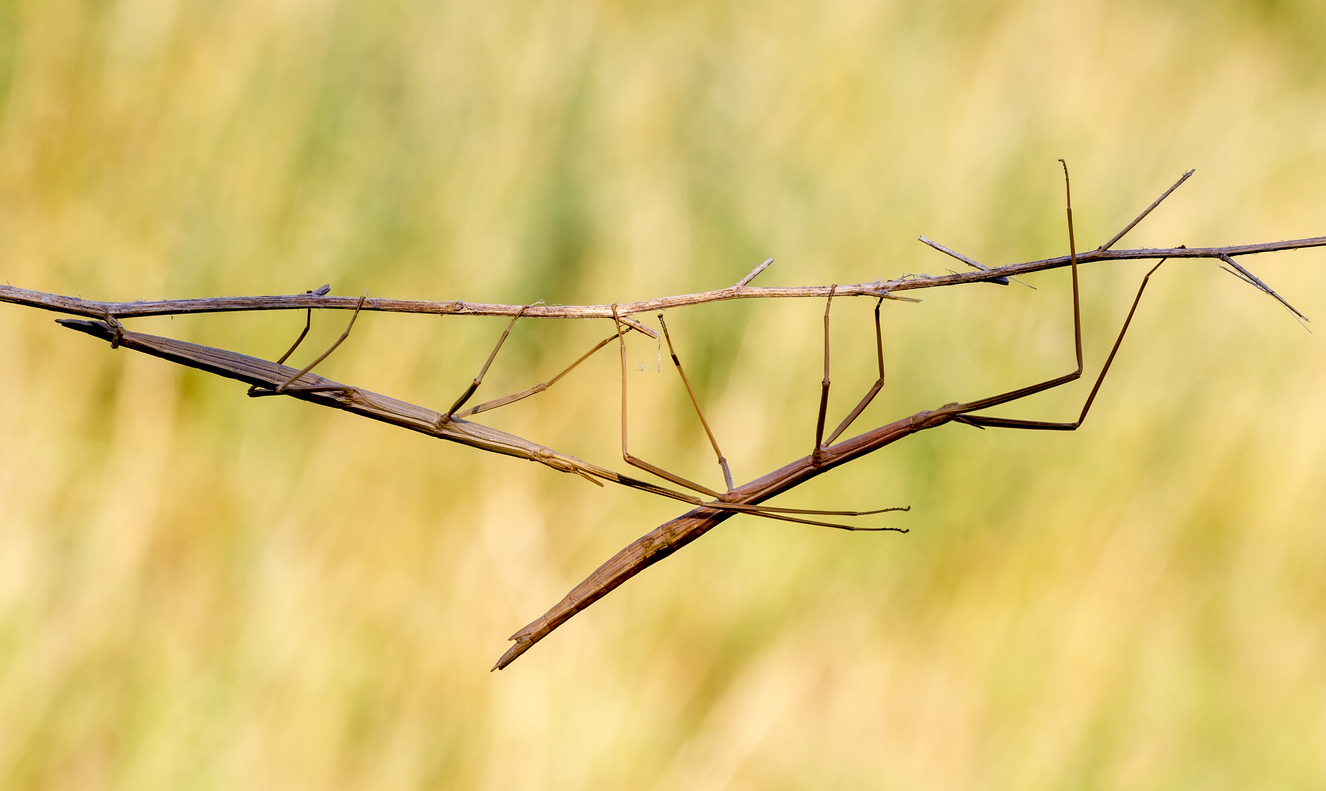This is a professionally taken, close-up, full-color photograph of two stick bugs camouflaged on a thin, bare branch, shot outdoors in natural daylight. The horizontally rectangular image uniquely captures the elusive nature of these insects, which blend seamlessly into the branch due to their brown, twig-like appearance. Located approximately just inside the left edge and extending across the frame to the right edge, the branch serves as a stage for these masters of disguise. The larger bug is on the right, with its six slender legs curling around the branch, while the slightly smaller one is positioned more towards the left, similarly gripping the branch with its six legs. Their antennae and body contours are subtly visible, suggesting their presence through the angles and curvature of their legs. The background is entirely out-of-focus, featuring a blurred mix of greens, yellows, and tans, likely indicative of surrounding vegetation, which helps draw the viewer's attention to the intricate details of the camouflaged insects.